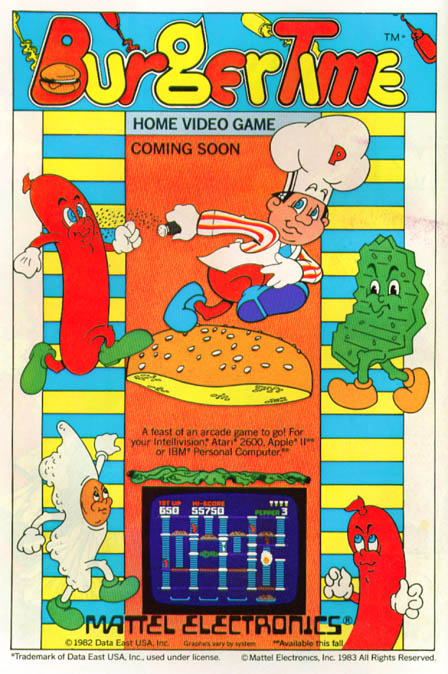The image appears to be the cover art for the video game "Burger Time." The design is vibrant and whimsical, featuring a palette dominated by light blue, light yellow, bright red, and various shades of green. At the top of the cover, the title "Burger Time" is prominently displayed in bold red and yellow letters against a blue backdrop. Directly below the title, in black text, it reads "Home Video Game," with the words "Coming Soon" right underneath that in the same style.

The central area of the cover is vertically oriented and features an orange rectangular section. Within this section, a colorful illustration captures immediate attention. The scene depicts a cartoon chef character energetically running across the top bun of a burger, which is orange on the outside with yellow on the underside, complete with sesame seeds. To the left of the chef, a red hot dog character is shown, sporting green shoes and white fists, suggesting it might be a quirky adversary or obstacle in the game. On the right side, a green character, which appears to be a piece of lettuce or a pickle, is wearing brown shoes, adding to the playful and imaginative design of the artwork.